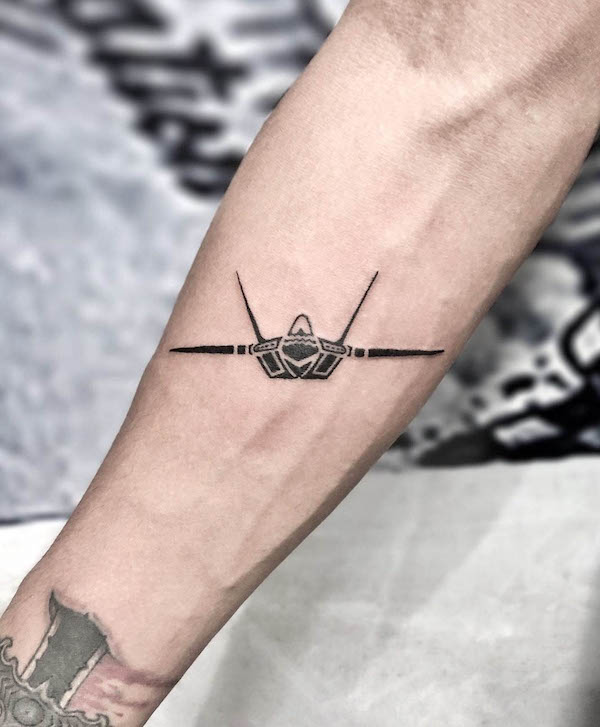This is an indoor, color photograph featuring a close-up of an adult white male's forearm, angled from the lower left to the upper right corner of the image. The background is a blurred, black-and-white or gray tone, making it difficult to discern any details, but it suggests either a rough-surfaced wall or a t-shirt. The forearm, appearing veined and fairly muscular, displays two tattoos. The prominent mid-arm tattoo is a relatively simple design in black ink, resembling a spaceship or fighter jet with thin, black antennas and wings. This design has an egg-shaped top with a parallel body structure, using minimal intricate details. Near the wrist, there's an older, faded tattoo that vaguely resembles a sword with blood drops, partially piercing the skin.